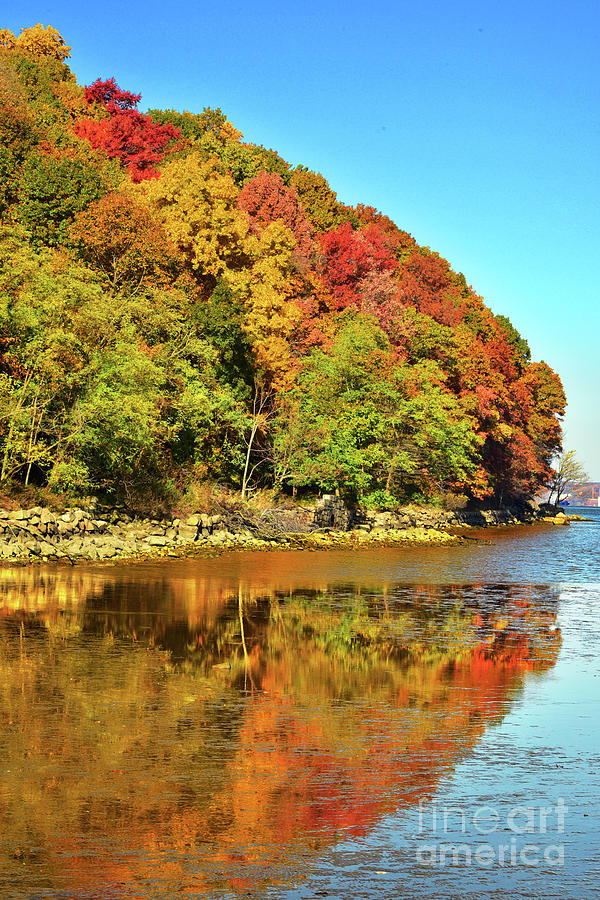The image is a detailed photograph capturing a serene river scene in the fall. The composition reveals a large, tree-covered landmass on the left in the background, showcasing a variety of autumn colors. The trees on the left transition from light green at the bottom to darker green at the top, with a section in the center featuring vibrant golden yellows and touches of red. On the right side, a single green tree stands out among a mix of reddish and orangish foliage.

The rocky shoreline, composed of yellow rocks, extends along the middle of the image, where a few people can be seen walking in the distance. In front, the river's surface appears brownish but may actually be reflecting the myriad colors of the trees. The water close to the viewer is vividly green due to the reflection of the surrounding trees. The sky occupies the upper half of the photograph and is a clear, deep blue without any clouds.

Additionally, there's a noticeable watermark in the lower right corner of the image, which is whitish and reads "Fine Art America." The sharp contrast between the vibrant fall colors and the clear sky adds to the captivating beauty of this autumnal river scene.